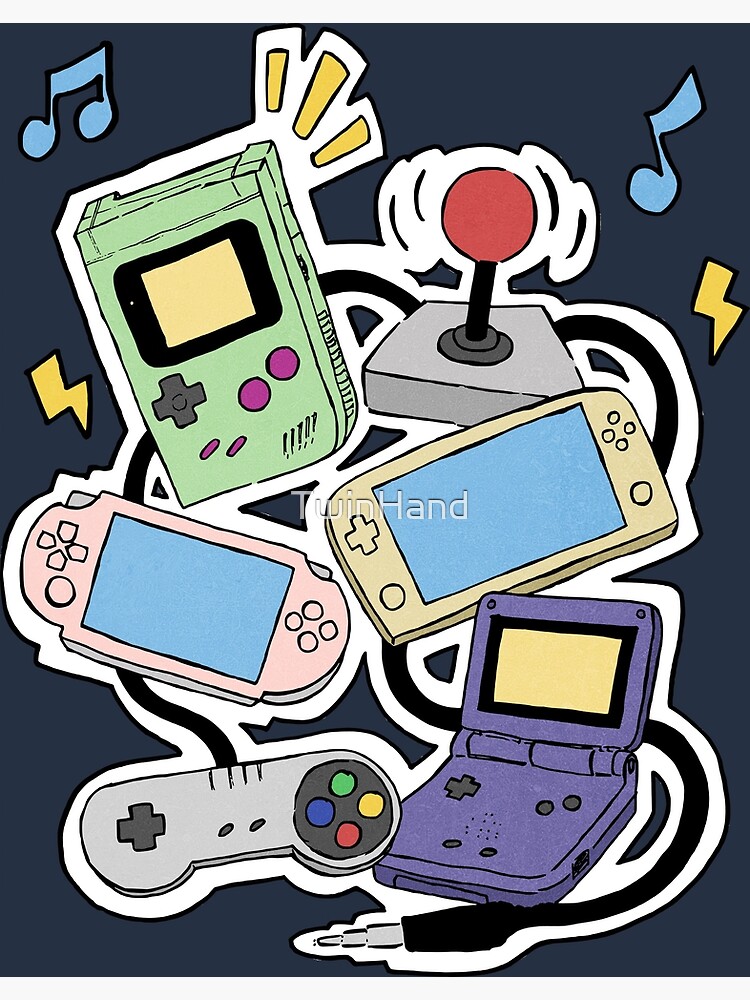The image is a detailed cartoon illustration reminiscent of early 2000s to early 2010s artwork, featuring various video game devices and elements on a dark blue background. Central to the image are multiple gaming controllers and handheld systems, all interconnected by a black rope-like cable ending in an auxiliary jack connection. At the bottom, a silver and gray controller is depicted, with a circular black area on one side containing colored green, yellow, red, and blue buttons, and a gray cross on the other side. Adjacent to it, there's a purple handheld device with a screen that folds up. In the middle, a green handheld game system resembling a Game Boy stands out with darker green or dark gray control buttons and two round pink buttons on the side. Nearby, a red joystick with a circular ball top and black stick is positioned on a light gray base. Two identical handheld devices with blue screens and pink and gold bodies, respectively, are also visible. The top of the print is adorned with colorful musical notes and yellow lightning bolts, adding a dynamic and nostalgic touch to the overall composition.